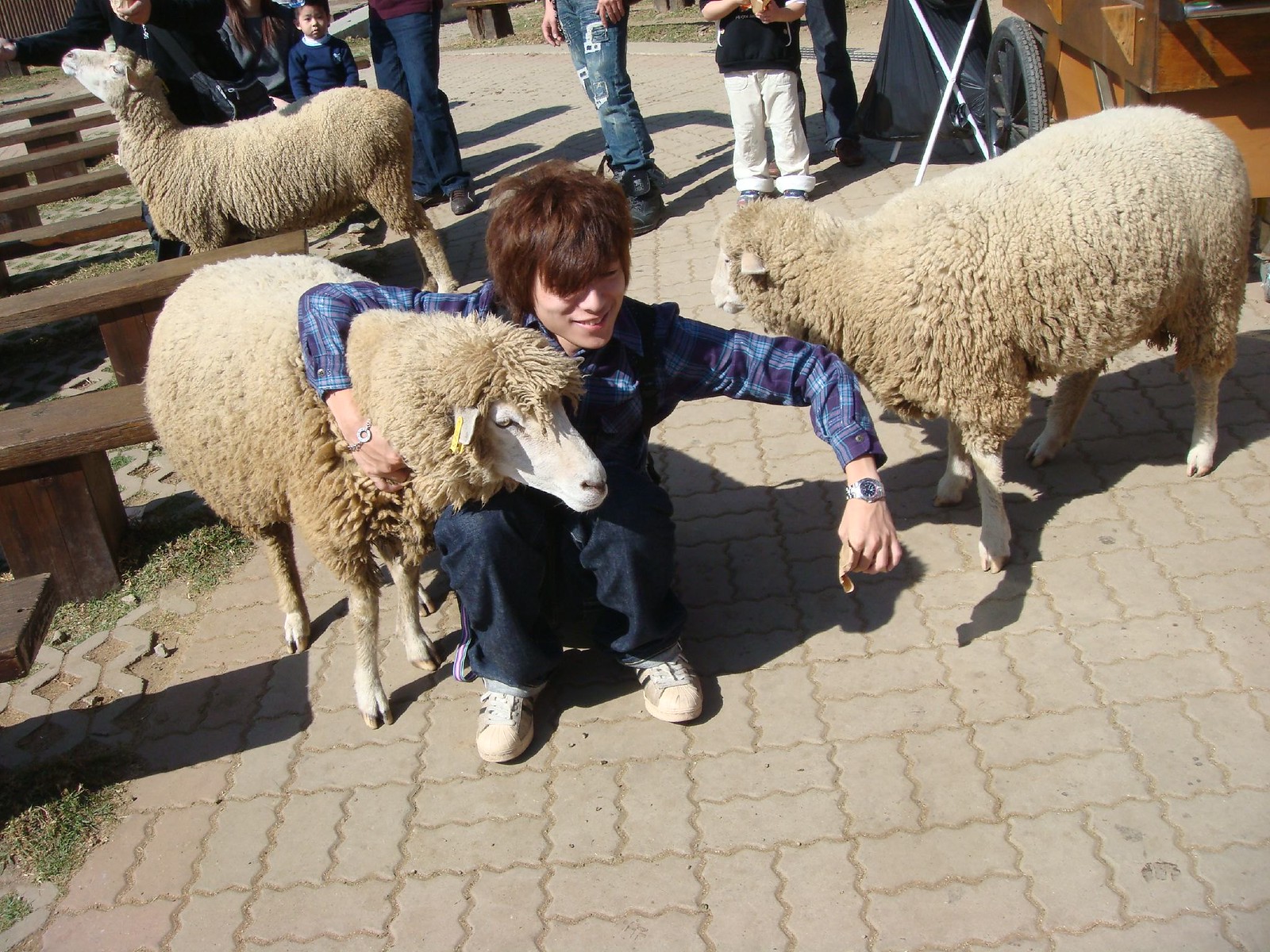In an outdoor setting that appears to be a petting zoo, a young boy, who looks to be around 12 or 13 years old, is squatting down on a ground paved with erratically shaped tiles that have curly borders. He has long, shaggy brown hair and is dressed in a blue and purple plaid long-sleeved shirt, blue jeans, and white tennis shoes. The boy is wearing a wristwatch and smiling as he interacts with two lambs. One lamb is nestled under his arm while the other stands beside him, facing away. In the background, there are wooden benches and a possible wagon or cart to the right of the photo. Various adults and children, mostly visible only from the waist down and dressed in jeans and pants, stand around, adding to the family-friendly atmosphere. The lambs, some of which have tags on their ears indicating they belong to a managed herd, seem tame and comfortable among the visitors.